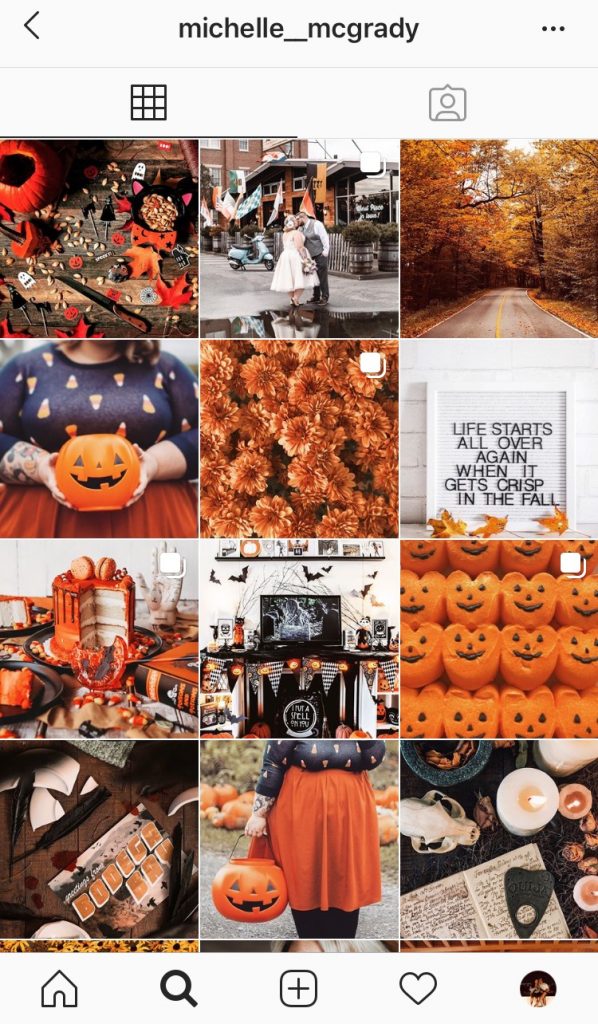The screenshot shows a mobile phone displaying a Pinterest page belonging to "Michelle_McGrady." At the top of the screen, a white bar with black text features the username "Michelle_McGrady." On the left side of the bar, there is a small black back arrow, and on the right side, three black dots are aligned vertically. Beneath this bar is a faint black line.

Below the line on the left, there is a black 3x3 cube icon, and to its right is a gray chat bubble icon containing a human head silhouette. The main content underneath these icons displays a Pinterest feed consisting of four vertical rows of three images each, all themed around Halloween pumpkins.

In the upper-left image, a small pumpkin appears to be in the process of being carved. The image to the right of it depicts the exterior of a restaurant with what looks like a ghost decoration hanging outside. The third image in the top row shows a road flanked by vibrant fall foliage. 

In the second row, the leftmost image features an overweight woman wearing a candy corn-themed T-shirt and holding a plastic pumpkin in her hands. The remaining details of the images are not described, but the visible items support the Halloween and autumn theme present throughout the Pinterest page.